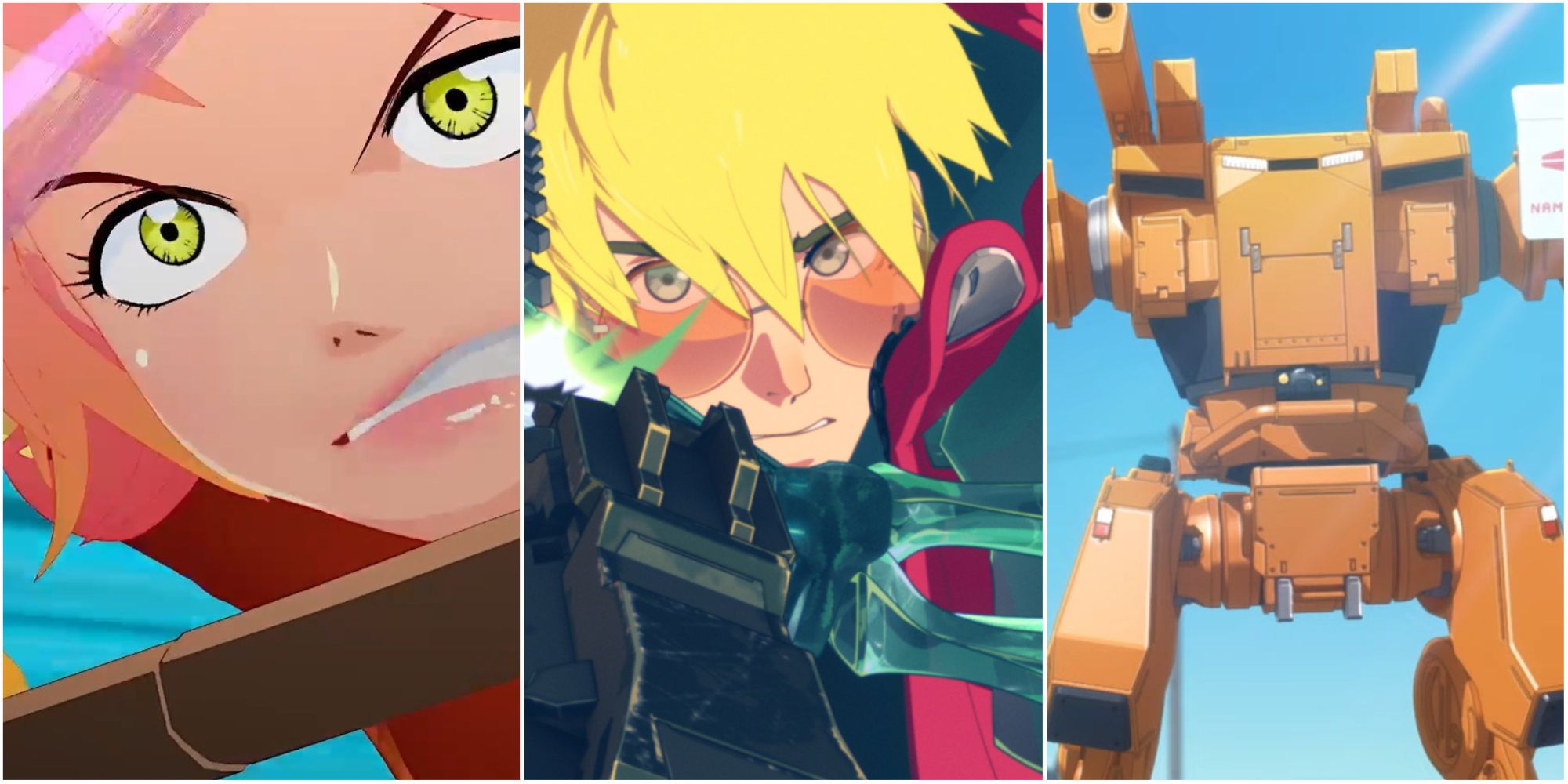This horizontally rectangular image is comprised of three vertically rectangular anime-style pictures, separated by white vertical lines and set against blue backgrounds. The leftmost image features an up-close shot of a young woman with a fierce, determined expression characterized by gritted teeth and a focused snarl. She has large green eyes with yellow undertones, white skin, and purplish-orange hair. Wearing rust-colored clothing, she appears to be gripping something in front of her, possibly a sword sheath.

The central image depicts a blonde-haired man with blue eyes, clad in a pink outfit and sporting distinctive circular glasses. He holds an indeterminate black object, potentially a weapon, which is partly obscured due to the close-up nature of the shot.

The rightmost image showcases a rust-colored robot standing on two legs against a light blue sky. The mechanoid displays a gun mounted on its left shoulder, though its arms are not visible. Despite its robotic appearance, it maintains a humanoid form, adding a dynamic, technological contrast to the other characters.